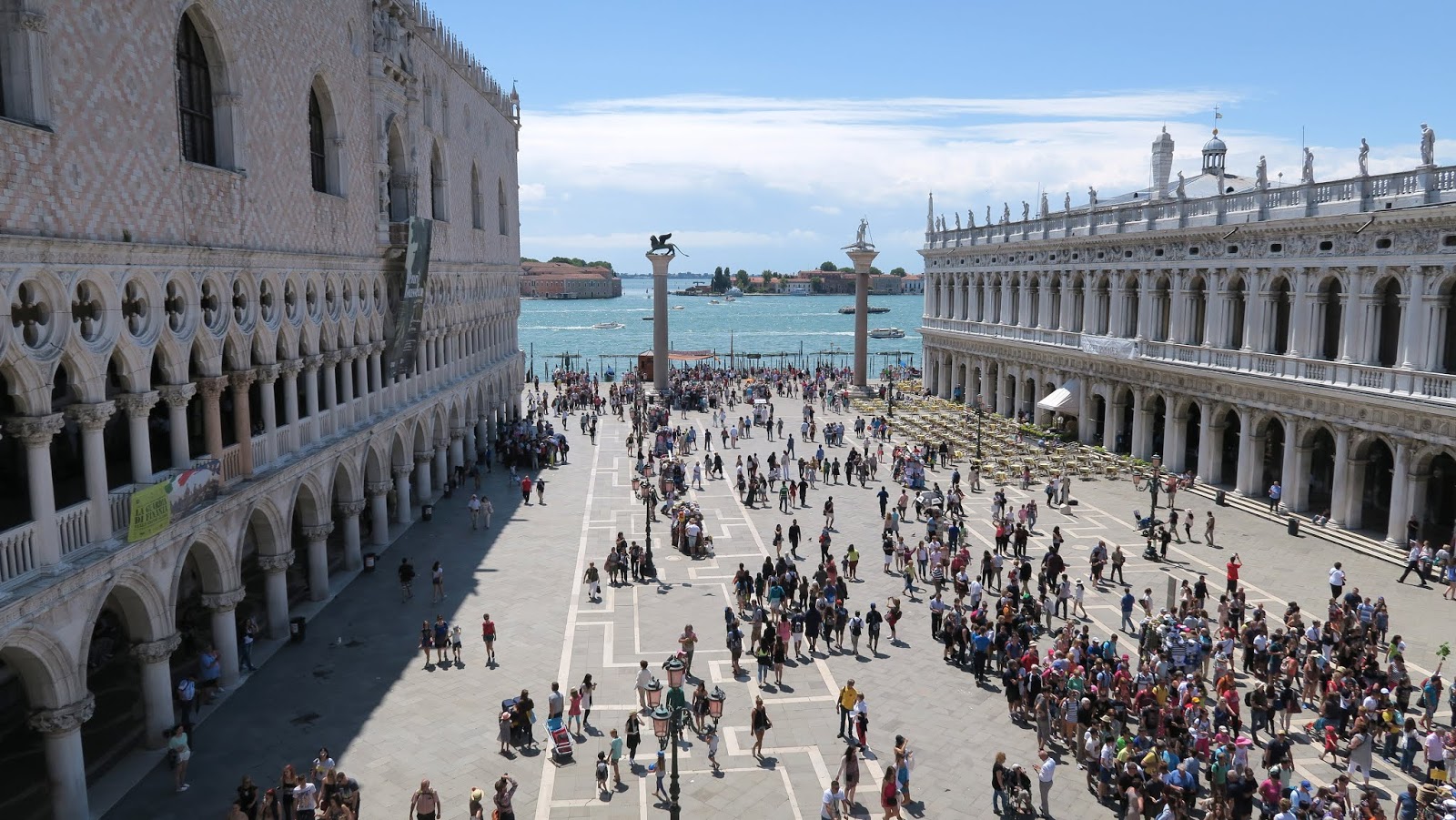The full-color photograph captures an outdoor scene on a bright sunny day, illuminated by natural light with some areas in shade. The setting is an expansive, bustling courtyard situated between two stately, government-like buildings. The building on the right is a two-story, white structure adorned with ornate columns and statues adorning its top story. On the left is a three-story, ornately designed stone building featuring numerous columns as well. Both buildings have arches on their lower levels that cover walkways and display banners attached to some of their pillars.

The courtyard itself is filled with groups of people, tourists predominantly, either milling about or standing in designated lines marked on the ground. There are also chairs set outside one section of a building. The image is taken from a top angle, providing a broad view of this open area where the crowds converge.

Above the courtyard, the sky is a clear blue dotted with some clouds, and below this, in the distance, is an enticing body of water with several boats sailing back and forth. Off in the distance, you can see islands with structures and greenery, completing this vivid, lively outdoor scene.